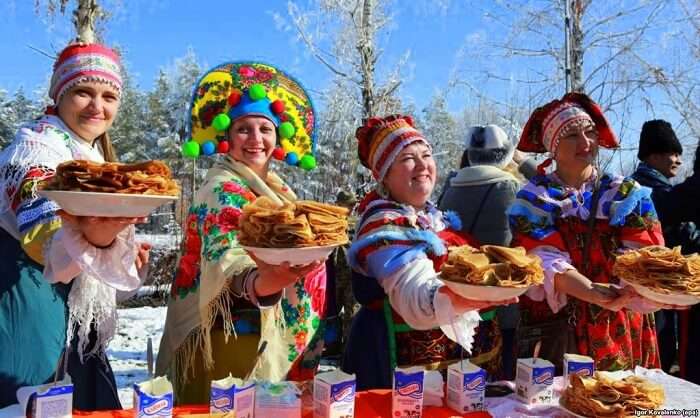This photo captures a lively outdoor winter celebration, evident from the snow covering the trees and ground. The event appears to be a traditional European festivity, as participants don cultural attire that includes colorful handmade scarves and beanies. In the foreground, four women are dressed in these traditional outfits, with one notably wearing a distinctive yellow hat adorned with ball-like decorations. Each woman holds a plate of food—possibly lightly folded pancakes—while standing before a table laden with an array of dishes and several opened milk cartons, presumably used in the food preparation. The joyous atmosphere and traditional garments suggest a festive occasion rich in cultural heritage and culinary delights.